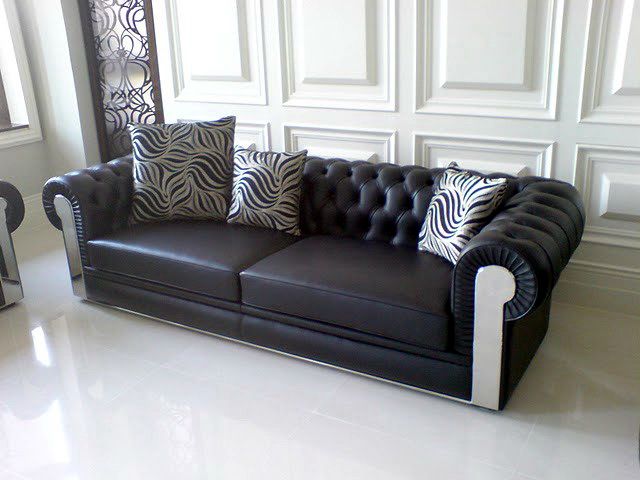This image showcases a luxurious living room space dominated by an elegant, long couch made of very dark blue or black leather material, featuring white accents on the armrests that extend to the floor. The couch, with a contemporary low-back design, is adorned with three high-end pillows that exhibit intricate patterns in white and matching blue hues, or in a swirly, wavy black-and-white design, adding a sophisticated touch. The room itself is predominantly white, with polished white marble flooring and a recessed, rectangular paneled wall that frames the scene with an air of opulence. In the corner behind the couch stands a wine rack or decorative metal shelf, contributing to the upscale ambiance. To the far left, there is a partial view of another similar armrest and a window with a white frame and a possible black ledge or sill, hinting at the spaciousness and elegance of the room. The overall composition evokes the feel of a high-end advertisement display, showcasing the couch as the centerpiece of this beautifully styled, wealthy-looking living area.